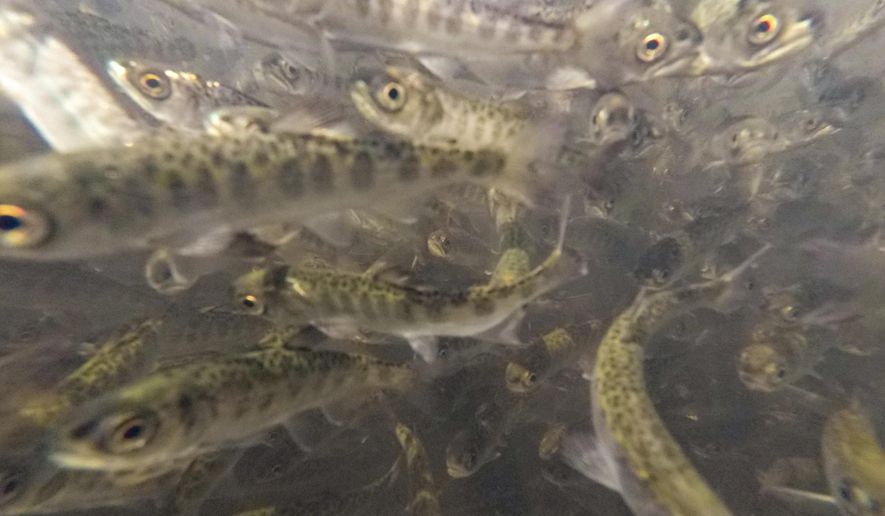The image captures a dense school of baby salmon swimming upstream, likely taken with an underwater camera. There appear to be at least a hundred salmon in the frame, each characterized by their long, slender bodies. The fish exhibit a light brown hue on their undersides, contrasted by darker brown and gold spots on their upper bodies. Their eyes glint with a distinctive gold tint. While most of the salmon are swimming forward, there is one in the center that is veering to the right. Despite the proximity of the camera, the fish remain undisturbed and continue their rapid movement, as evidenced by the blur of their fins. The detailed shot allows for a clear view of their intricate patterns and streamlined forms.